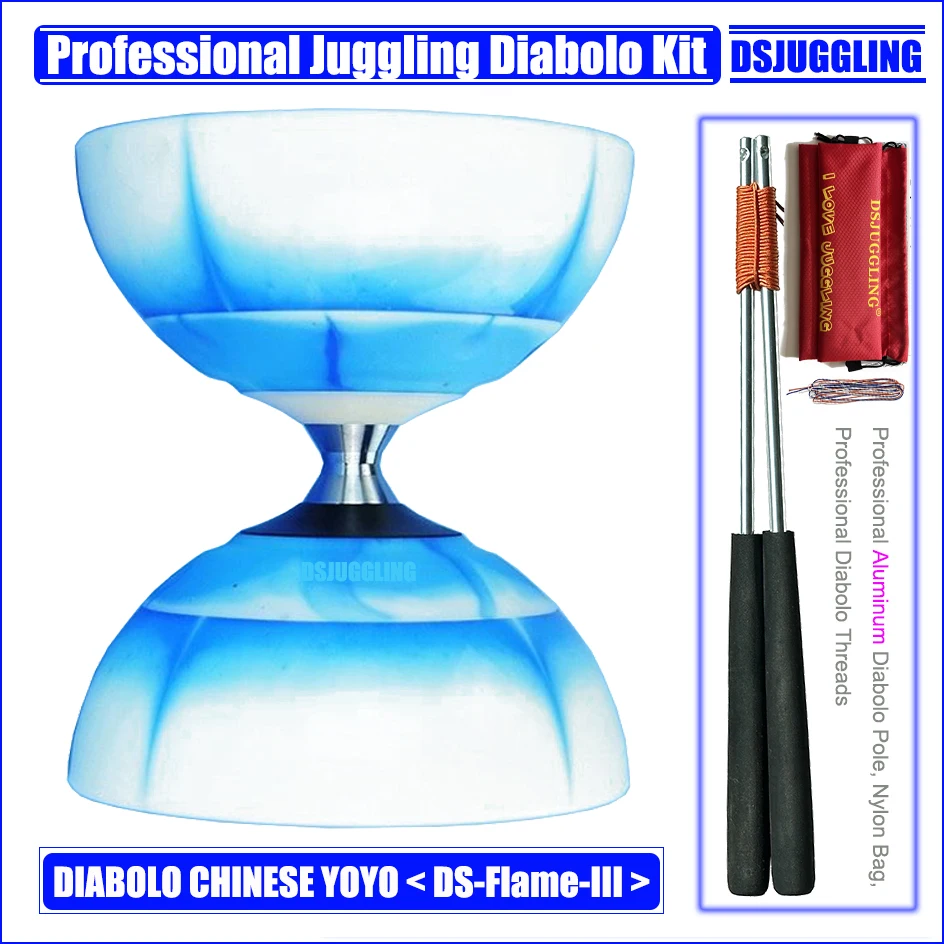This color photograph is a detailed advertisement for a Professional Juggling Diablo Kit—a Chinese yo-yo set. At the top of the image, a bright blue banner features bold white text that reads "Professional Juggling Diablo Kit". On the right side, "DS Juggling" is emblazoned, while at the bottom, another blue bar contains white text that says "Diablo Chinese Yo-Yo DS Flame 3".

At the center of the image is the primary component of the kit: the diablo itself. This diablo comprises two large, bowl-shaped sections, resembling upside-down igloos or chalices, connected by a silver center spindle. The upper and lower sections of the diablo feature light blue and white coloring with distinctive blue streaks. The colors of the collars differ between the sections, with one being white and the other black.

To the right, the kit includes additional accessories for the diablo. These include two metal poles with black padded handles and silver tips, connected by a rope at the top. Adjacent to these poles is a red nylon storage bag featuring "I love juggling" text. Another set of text within this right-hand section lists the accessories as "Professional Aluminum Diablo Pole, Nylon Bag, Professional Diablo Threads."

The detailed presentation of items and supportive elements in vibrant blue, black, red, and gold hues, gives potential buyers a comprehensive view of the juggling kit's components and their professional-grade construction.